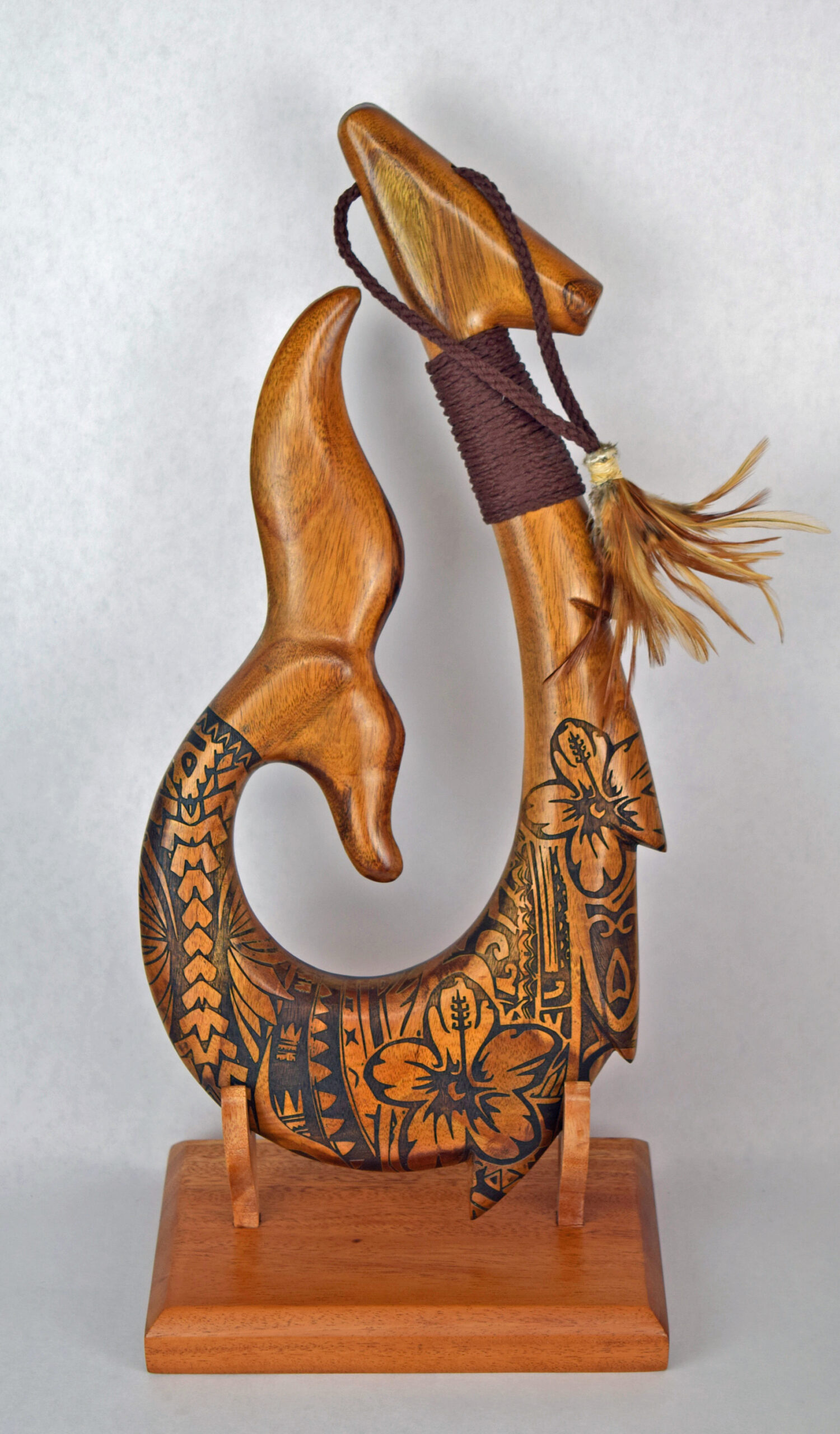The image captures a detailed indoor photograph featuring a unique ornamental object. The background is a gradient gray, seamlessly blending from the wall into a solid gray shelf. On the shelf rests a wooden platform with beveled edges, supported by two raised holders. The centerpiece is a meticulously carved wooden sculpture resembling a hook. The object, about six inches high and three inches wide, features intricate details suggestive of a maritime theme. At the top, a cord is attached, holding a brown feather. Further down, the handle is wrapped with cord, adding texture.

As the sculpture curves, the hook’s right side spikes slightly, adorned with designs reminiscent of Maori or Polynesian art. These intricate black patterns include hibiscus flowers and geometric shapes. The hook curves gracefully to form a point resembling a whale’s tail. The object is finished with ornate, tattoo-like designs in dark blue and greenish hues, enhancing its exotic appearance. The entire piece is balanced on the wooden stand by its two leg-like extensions, creating a stable display. The exact nature of the sculpture is ambiguous, blending elements of a fish fin and hook, evoking a sense of cultural artistry.